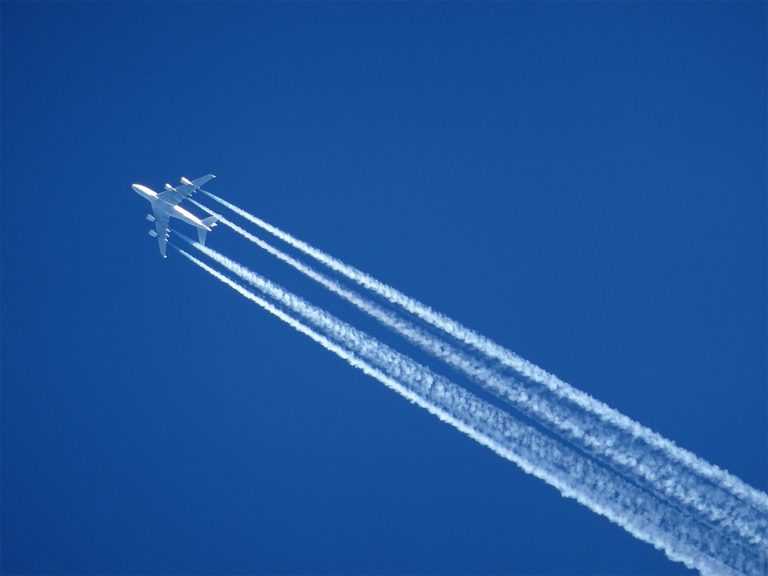The image captures a large, white jet airliner flying diagonally across a deep, crystal clear blue sky from the lower left to the upper right. Seen from the ground, the jet’s four substantial engines, mounted on swept-back wings, are clearly visible. The plane is trailing four long, straight contrails that cut impressively through the sky, resembling the wake of a boat skidding across a calm lake. There are no markings, text, or colors other than the clean, silverish-white of the jet and its contrails. The sky's rich blue suggests that the photo was taken either early in the morning or late in the evening, as it’s deeper and darker than midday sky. No other elements are present to distract from the jet and its striking trails.